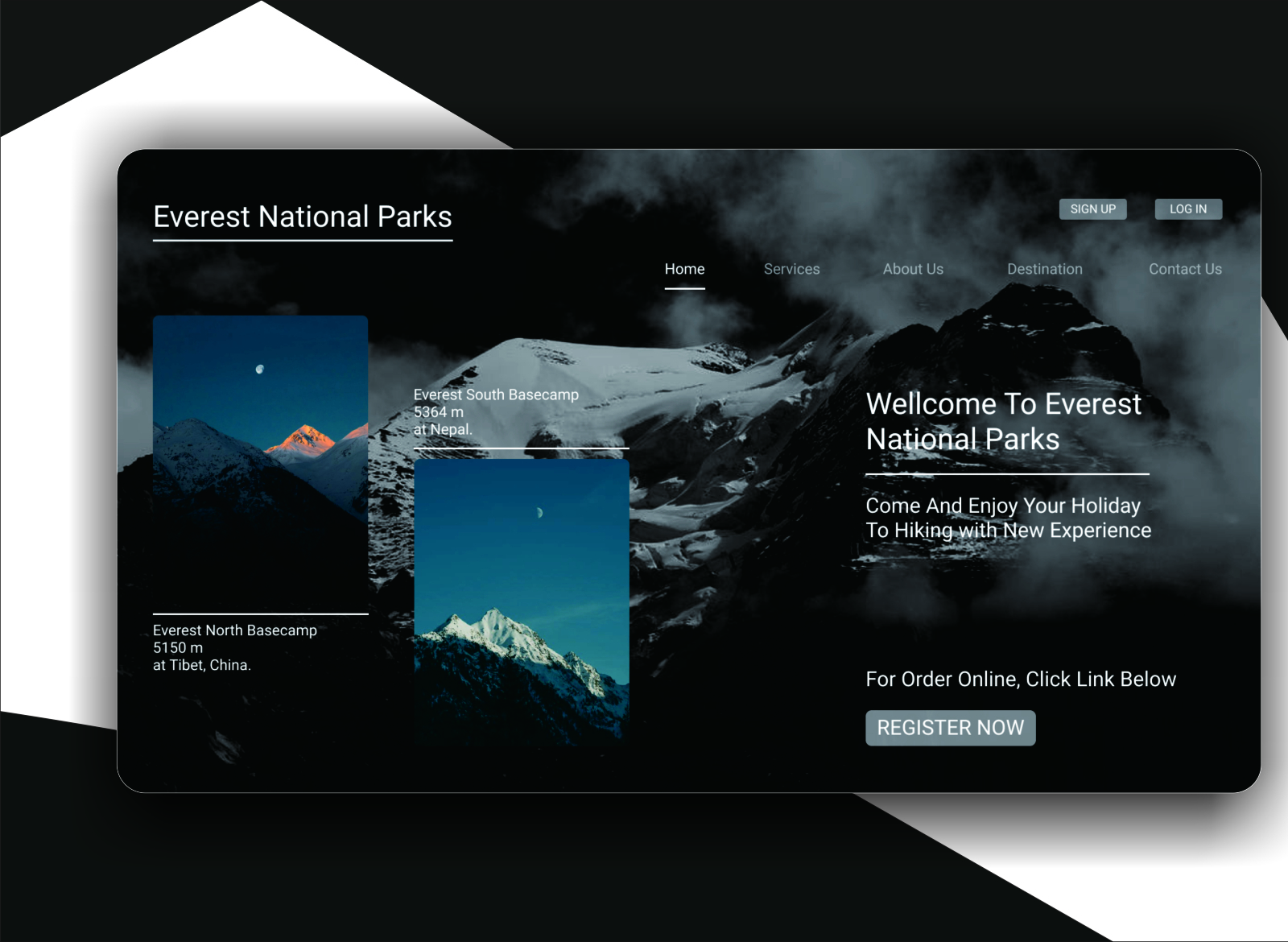Here is a detailed descriptive caption for the image:

"Screenshot of an informational webpage about National Parks at Mount Everest in Nepal. The image has a wider-than-tall aspect ratio and features a black-and-white background. At the center, there is a rectangular element with rounded corners and a dark overlay, reminiscent of a credit card. Superimposed on this overlay are misty images of Mount Everest's majestic peaks. Prominent labels identify key locations; Everest North Base Camp at an altitude of 5,150 meters in Tibet, China, and Everest South Base Camp at an altitude of 5,364 meters in Nepal. The text on the overlay invites viewers to 'Welcome to Everest National Parks,' encouraging them to 'come and enjoy your holiday hiking with new experience.' Additional text offers instructions for online orders and encourages registration with a 'Register now' prompt, followed by navigation options like Home, Services, About Us, Destination, and Contact Us. Though it uses official-sounding language suggesting governmental affiliation, the webpage appears to promote a commercial venture specializing in guided hiking tours to Everest, providing services for hire rather than operating as a government-run institution."